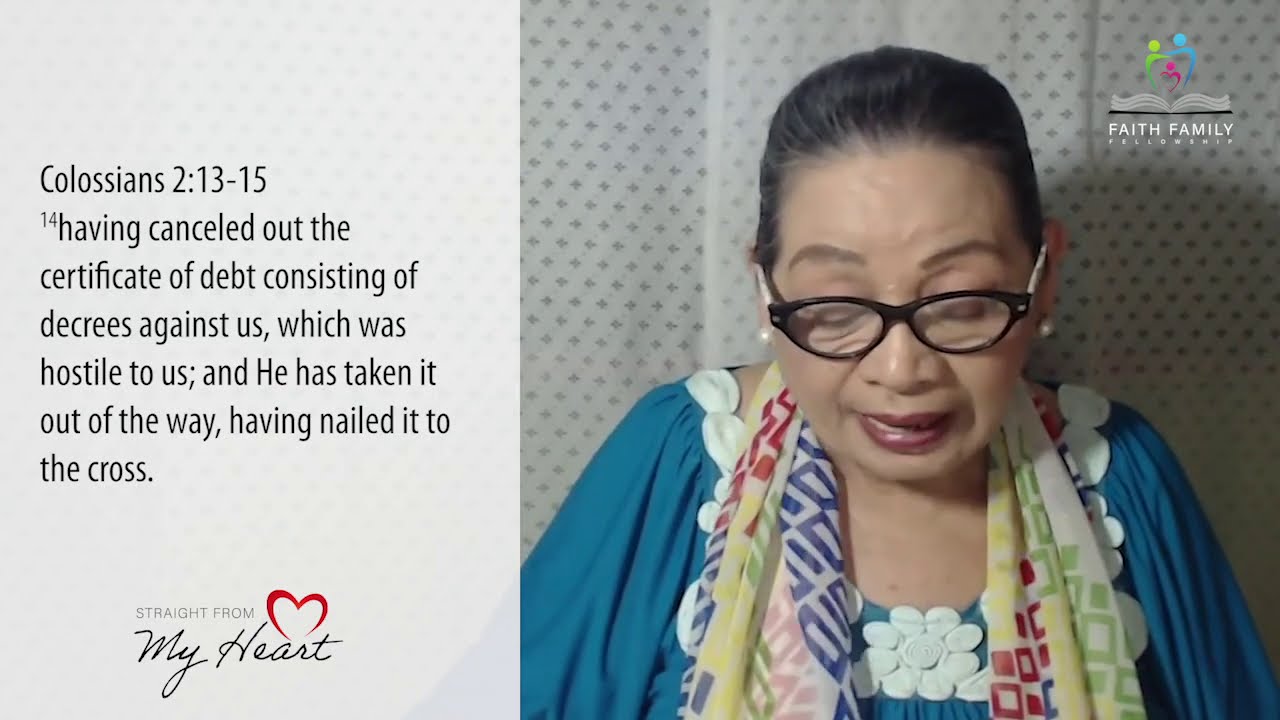The image features an elderly woman, approximately 50 years old, with black hair and glasses, dressed in a blue dress and a colorful, flower-patterned scarf in shades of blue, green, pink, yellow, and red. She is gazing downward, and behind her is a white wall with a gray textured pattern. On the left side of the image, there is a white transparent box containing a biblical quote from Colossians 2:13-15, which reads: "Having canceled out the certificate of debt consisting of decrees against us, which was hostile to us, and He has taken it out of the way, having nailed it to the cross." At the bottom of the image, the phrase "Straight from my heart" appears alongside a small red heart logo. The top right corner features the words "Faith Family Fellowship" next to an open book with three people depicted within it, suggesting this is an advertisement for a church or religious group on social media.